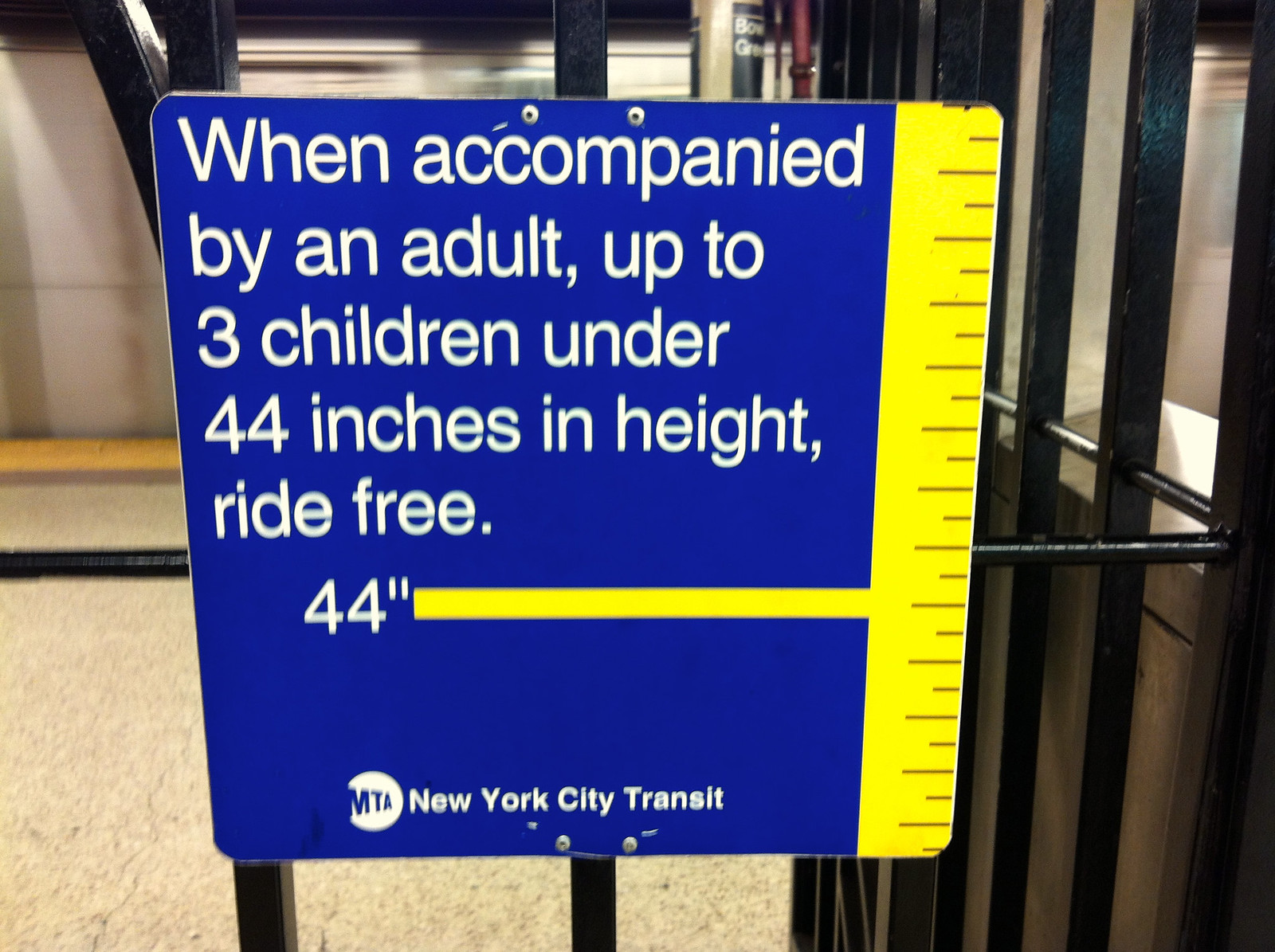The photo depicts a detailed scene in a New York City Transit subway station. Central to the image is a blue sign affixed to black metal bars. The sign features a yellow ruler on its right side, highlighted by a yellow mark at the 44-inch height. The text on the sign states, "When accompanied by an adult, up to 3 children under 44 inches in height ride free.” Below the text, the MTA New York City Transit logo is displayed in white. The sign allows children to measure their height against the ruler. The background reveals the typical subway environment with concrete flooring, visible black railings, and a platform with a notable yellow safety line at its edge. Pillars and the presence of the subway tracks are subtly visible, enhancing the urban transit setting.